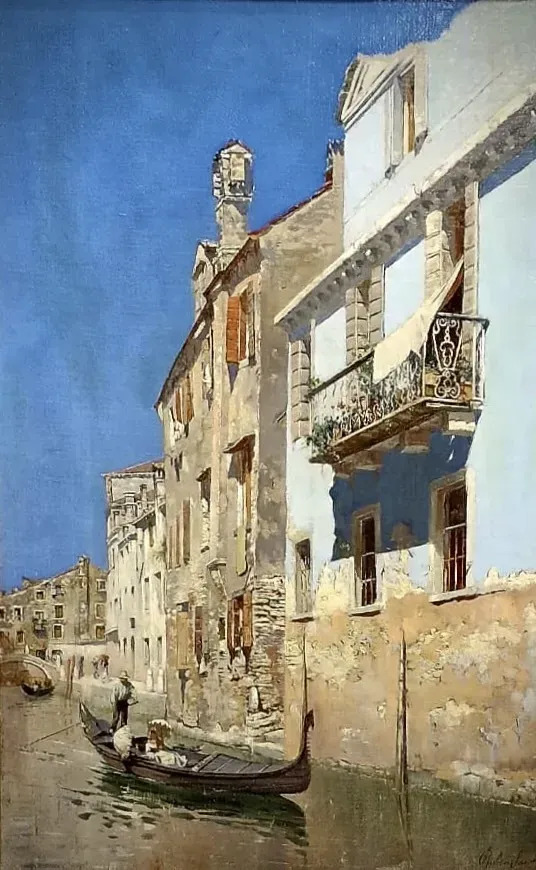The image beautifully captures a serene canal scene, possibly set in Italy, with an array of stone-built homes lining the water. The buildings are predominantly beige-brown, characteristic of the stone material, with one striking baby blue terrace that stands out. On the upper part of this terrace, a piece of clothing or a towel drapes over it, adding a touch of daily life to the idyllic setting. The sky is a vivid blue, contrasting against the earthy tones of the buildings and the grayish-green water of the canal. A small boat, likely a gondola, is positioned towards the right of the image. A man stands at the stern, steering, while a woman sits comfortably in the gondola, embracing the tranquil atmosphere. In the background, there's a glimpse of a bridge and another boat, enhancing the depth and charm of the scene. This picturesque and peaceful portrayal might be a painting or an AI-generated image, capturing the essence of a quiet day by the canal.